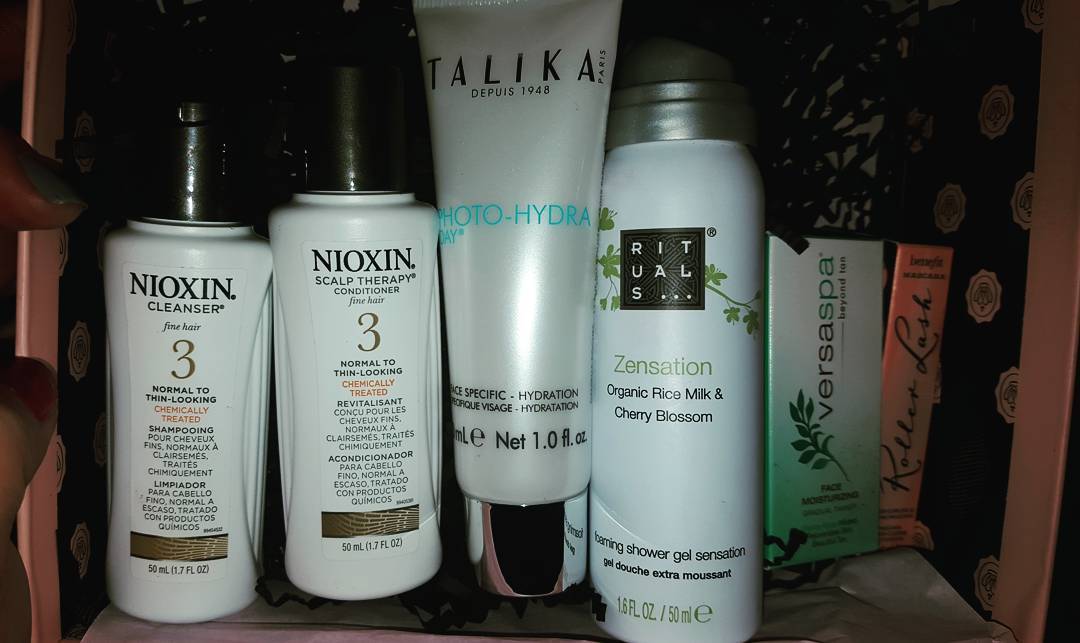This close-up image showcases a collection of beauty products arranged meticulously. Flanking the sides are shiny pink boxes with black interiors, creating a striking frame. On the far left, two fingers adorned with dark nail polish make a subtle appearance, although the exact shade is elusive due to the image's dim lighting.

Prominently positioned is a white bottle with a black lid labeled "Nioxin Cleanser." Its detailed description indicates it is suitable for fine, chemically treated, normal to thin-looking hair, with additional instructions provided in multiple languages. The bottle's bottom reads "50 milliliters."

Adjacent to the cleanser is another similar-sized bottle labeled "Nioxin Scalp Therapy Conditioner," also intended for fine, normal to thin-looking, chemically treated hair.

Adding variety to the ensemble, a longer tube with a silver cap stands below. It is identified as "Talika Photo-Hydra," containing 1.0 fluid ounces.

Complementing the collection is a white canister with a silver lid, labeled "Rituals Zensation" and detailing its contents: organic rice milk and cherry blossom foaming shower gel.

Interspersed among these bottles is a small white and green box labeled "VersaSpa," adding a touch of freshness to the scene.

On the far right, a tiny, vibrant orange box with the cursive inscription "Rolox Lash" completes the assortment of beauty essentials.

Each product is meticulously displayed, highlighting an array of skincare and haircare solutions.